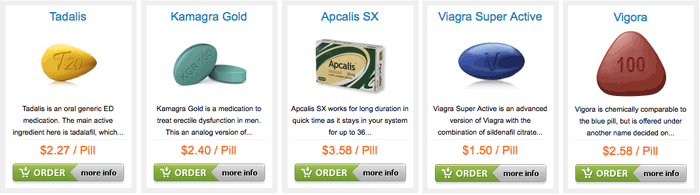Here is the cleaned-up and detailed caption for the image:

---

The image displays an assortment of five pills, each catering to male erectile dysfunction. Below is a detailed description of each:

1. **Tadalys**:
   - **Appearance**: Yellow pill
   - **Type**: Oral generic ED medication
   - **Active Ingredient**: Tadalys
   - **Price**: $2.27 per pill

2. **Camaragold**:
   - **Appearance**: Teal pill
   - **Type**: Analog version of an ED medication
   - **Purpose**: Used to treat erectile dysfunction
   - **Price**: $2.40 per pill

3. **Epicalis SX**:
   - **Duration**: Long-lasting effect, staying in the system for up to 36 hours
   - **Price**: $3.58 per pill

4. **Viagra Superactive**:
   - **Appearance**: Little blue pill
   - **Type**: Advanced version of Viagra
   - **Ingredients**: Combination of aldenafil and citrate
   - **Price**: $1.50 per pill (cheapest option)

5. **Vigora**:
   - **Appearance**: Brown pill
   - **Type**: Chemically comparable to Viagra, also known as the "little blue pill"
   - **Price**: $2.58 per pill

Note: The pill Epicalis SX, which is the most expensive at $3.58 per pill, had no specific color mentioned in the provided details.

---

This comprehensive description outlines the specific characteristics, active ingredients, prices, and purposes of each pill for easy identification and understanding.